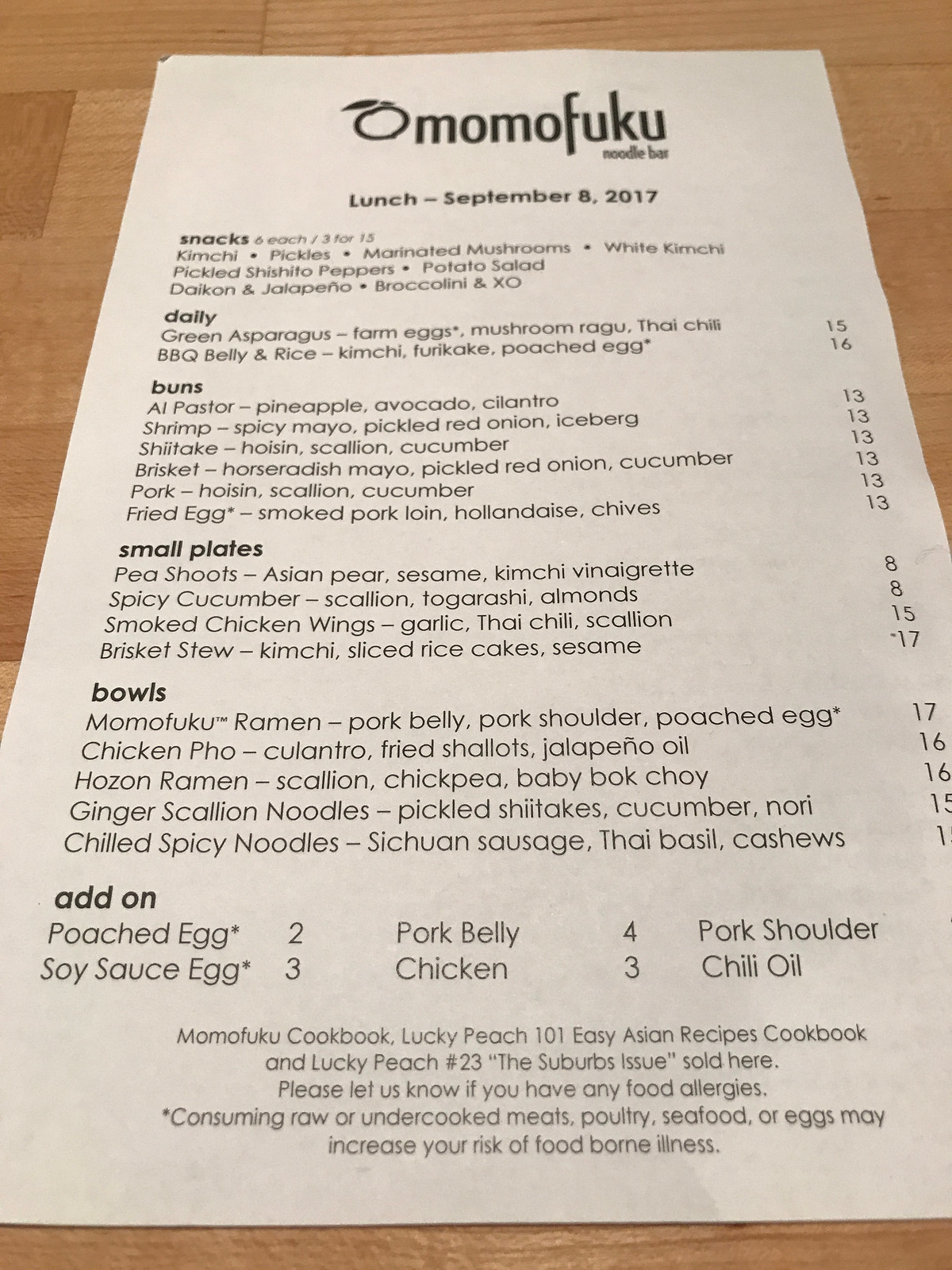This image features a menu from an Omamofuku Salad and Noodle Bar, presented on tan, parchment-like paper that is notably tall and narrow, at least twice as tall as it is wide. The text is rendered in black ink, with the title "Omamofuku" prominently displayed in bold black letters at the top, distinguished by the capital "O" while the rest of the letters are lowercase. Directly beneath the title, it states "lunch, September 8th, 2017."

The menu items are meticulously organized from top to bottom in a single column, categorized into sections labeled snacks, daily, buns, small plates, bowls, and add-ons. At the bottom of the menu, an additional message informs customers about Omamofuku's cookbooks— "Lucky Peach 101 Easy Asian Recipes Cookbook" and "Lucky Peach No. 23 The Suburbs"— available for purchase, and it includes a cautionary note about food allergies and the risks of consuming raw or undercooked meats, poultry, seafood, or eggs.

The prices, which are not explicitly confirmed to be in dollars, range from $13 to $16 for daily items, $13 for buns, and between $15 and $17 for bowls. The entire menu is photographed resting on a wood-grained, varnished light brown tabletop, adding a rustic touch to the setting.